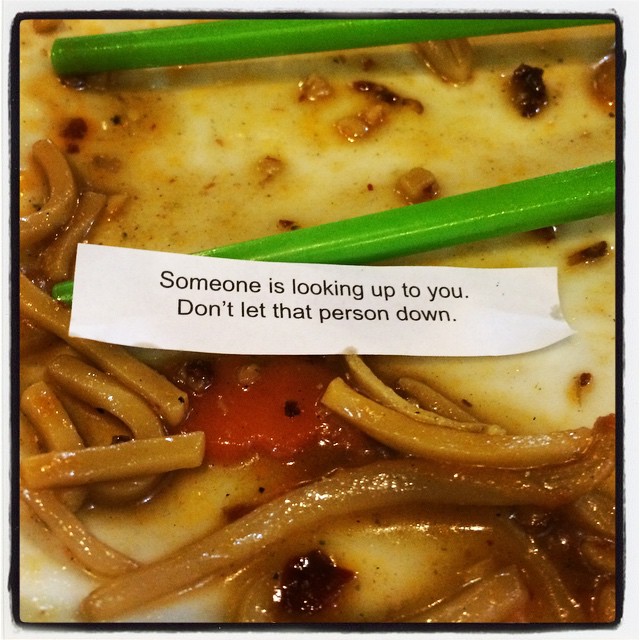The image depicts a partially eaten plate of Chinese food, characterized by a messy assembly of tan-colored noodles drenched in a watery, brown gravy-like sauce. Scattered throughout the plate are small cuts of vegetables, including a visible piece of carrot and perhaps some tomato with black specks, indicative of various spices. Two bright green chopsticks, positioned diagonally, are partially visible, hinting they might extend beyond the frame. Dominating the center of the image, atop the food, is a white strip of paper bearing a fortune in bold black text, stating: "Someone is looking up to you. Don't let that person down." The entire scene is framed by a black border, giving the impression of a candid shot of an unfinished, somewhat unappetizing meal.